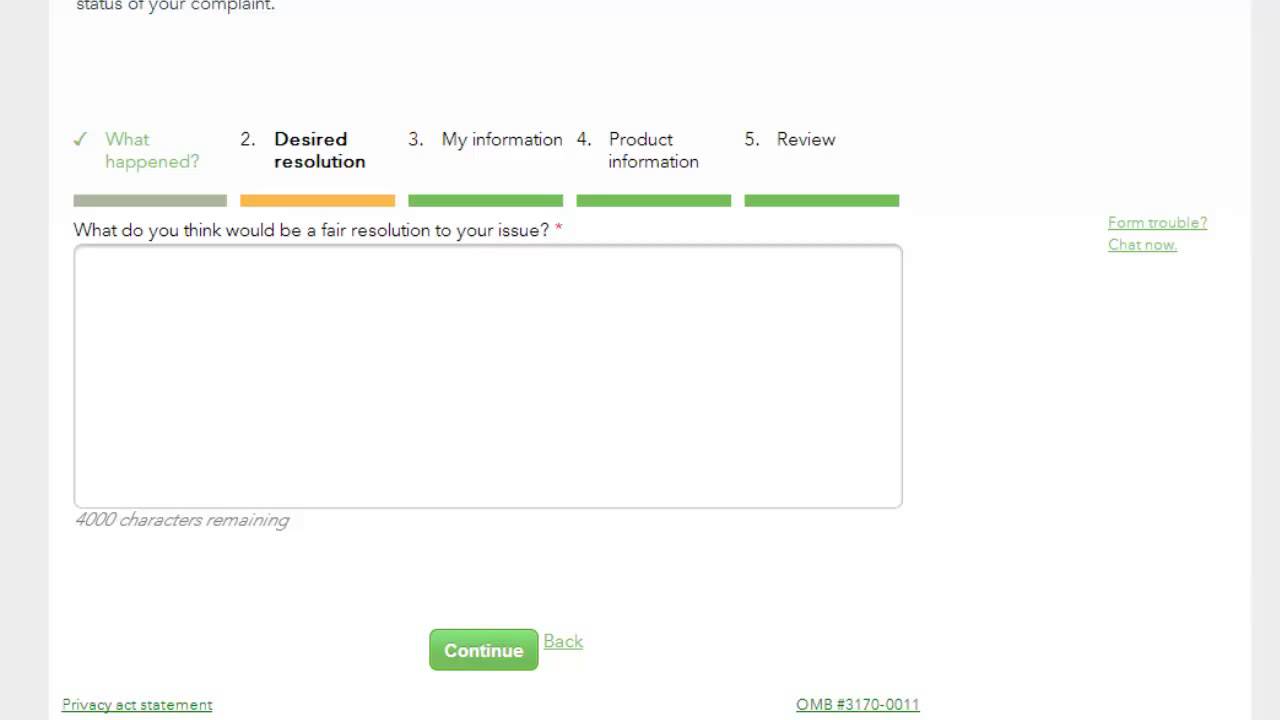The image is a rectangular form-oriented web page, displayed with its longer side stretching horizontally. The borders on the left and right sides are gray, framing the content within. The content background is white.

At the very top left of the image, partially cut off, it reads "Status of your complaint." Immediately below this header, there are several numbered sections indicating the steps of the complaint process:

1. **What Happened** - Highlighted with a green checkmark and accompanied by a gray bar beneath it, indicating it's the current step.
2. **Desired Resolution** - In bold black text and highlighted with an orange bar.
3. **My Information** - Less bold, marked with a gray bar underneath.
4. **Product Information** - Below this, a description in similar green bar styling.
5. **Review** - Followed by a corresponding green bar.

Beneath these steps, a prompt asks "What do you think would be a fair resolution to your issue?" This is followed by a gray outlined text box with a white fill, allowing space for a maximum of 4,000 characters, as noted beneath it.

On the right side of the box, there's a green underlined text reading "Form trouble? Chat now," suggesting an assistance link.

Towards the bottom center, there is a prominent green button with white text that says "Continue," and next to it, a green underlined "Back" option.

In the bottom left corner, there is another green underlined link labeled "Privacy Statement." On the bottom right, the text reads "OMB number 3170-0011," also in green and underlined.